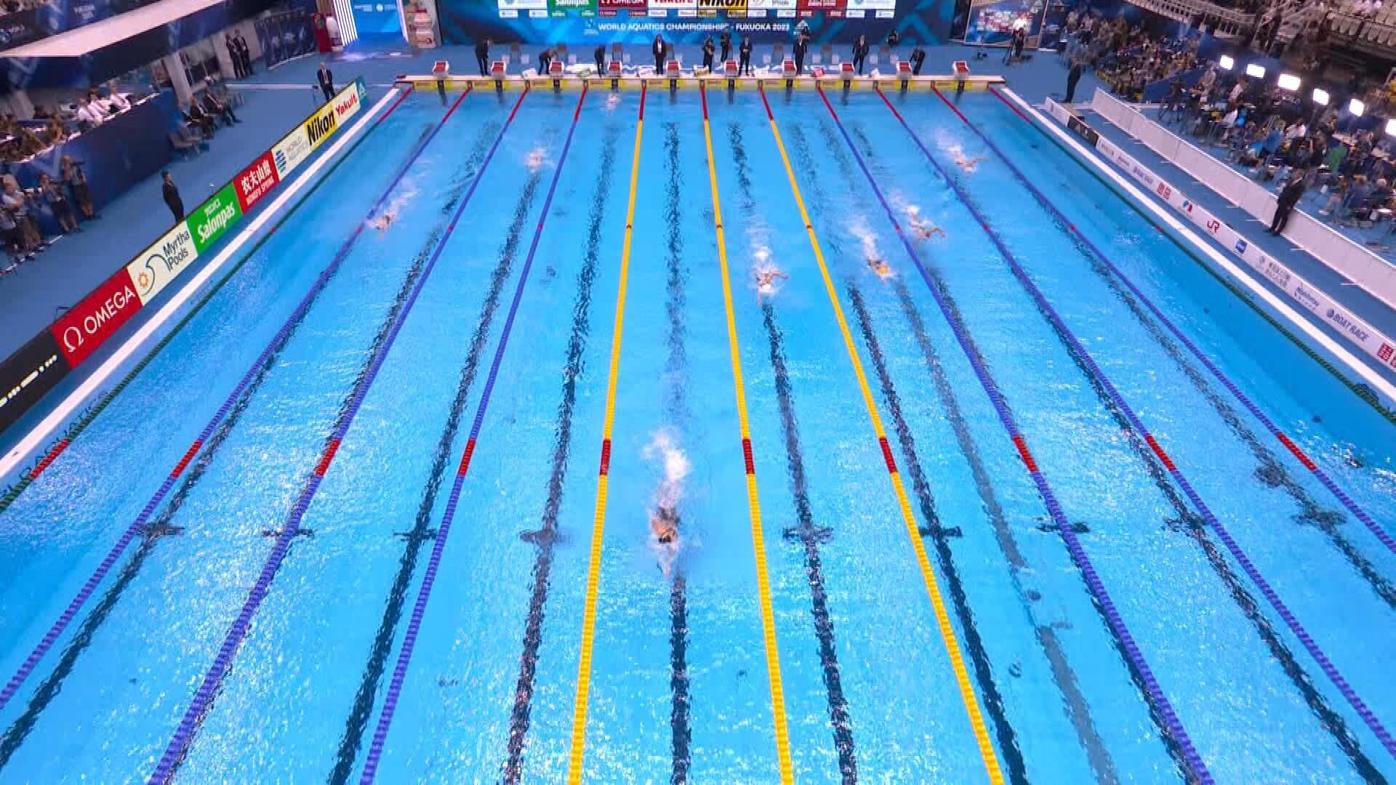This is an overhead photograph of an indoor swimming pool capturing the intense moment of a competitive race. The Olympic-sized pool is divided into ten lanes by alternating yellow and blue ropes, and each lane is occupied by swimmers at different stages of the race. The image captures a flurry of movement and splashing water, especially notable around the swimmer in the middle lane who is leading the pack. At the far end of the pool, there is a platform with judges positioned behind, overseeing the competition. Banners for advertising, including a prominent red one from Omega, line the sides of the pool. Powerful lights can be seen in the upper right corner, likely set up for television coverage. Spectators and possibly coaches or additional judges are seated or standing along the sides, adding to the vibrant and bustling atmosphere of the event.